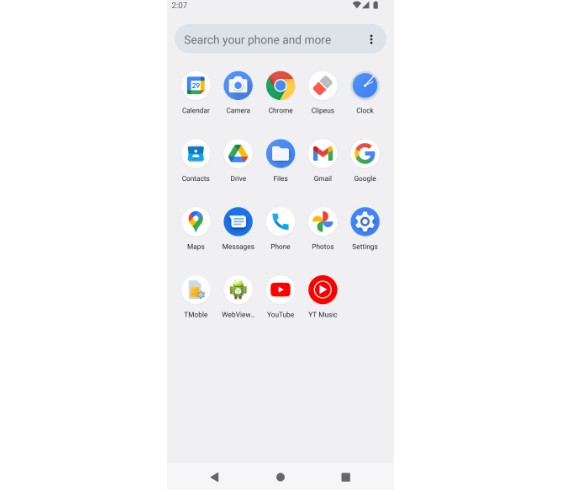This is a detailed photo of a smartphone home screen, likely an Android device, captured in portrait orientation. The image is approximately three times taller than it is wide. At the very top, the status bar displays a black font time reading "2:07" alongside icons indicating full Wi-Fi signal, full cell service, and a fully charged battery, all depicted in black.

Beneath the status bar, there's a search bar with a gray background that reads "Search your phone and more," suggesting it’s a comprehensive search function. Below this search bar are the main app icons arranged in a grid format of five columns and five rows, although the last row only contains four icons, making a total of 24 icons.

The icons visible include:

1. Calendar
2. Camera
3. Chrome
4. Clippus
5. Clock
6. Contacts
7. Drive
8. Files
9. Gmail
10. Google
11. Maps
12. Messages
13. Phone
14. Photos
15. Settings
16. T-Mobile
17. WebView
18. YouTube
19. YouTube Music

These apps predominantly consist of Google-related applications with a mix of other utility and personal apps, indicating a typical arrangement for easy access to frequently used functions on the device.